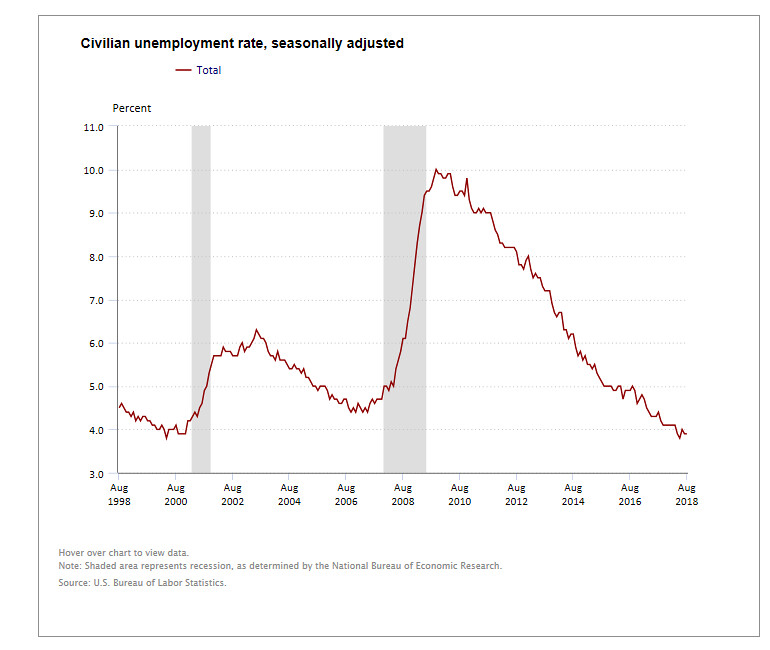The image depicts a line chart illustrating the seasonally adjusted civilian unemployment rate over a span of two decades, from August 1998 to August 2018. The title at the top reads "Civilian Unemployment Rate Seasonally Adjusted," with a legend below indicating that the red line represents the total unemployment rate. The y-axis on the left, labeled "Percent," ranges from 3.0% to 11.0%. 

The x-axis at the bottom charts years in increments of two, starting from August 1998 and ending in August 2018. Notably, the red line, which represents the unemployment rate, fluctuates over this period. It starts around 4.5%, dips slightly before rising towards August 2002, then decreases again by August 2007. However, it peaks sharply, reaching its highest point just before August 2010 at 10.0%, before gradually declining to around 4.0% by the end of the chart in August 2018.

Additionally, shaded gray areas on the chart denote periods of recession, as determined by the National Bureau of Economic Research. These shaded areas are particularly prominent between August 2000 to August 2002 and near August 2008. The bottom of the chart provides a note prompting the viewer to hover over the chart for detailed data, and the chart is sourced from the U.S. Bureau of Labor Statistics.